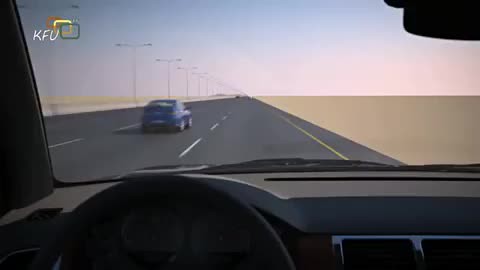This detailed description captures the essence of the scene from the image:

The image appears to be a screen grab from a video game showing the view from inside an American car, suggested by the left-side steering wheel. The dashboard is dark gray or black, featuring vents for the A.C. The windshield frames a multi-lane road made of black asphalt with white lane markings, and the car is driving on the right side. The scene outside shows a flat, sandy-colored expanse to the right and numerous utility poles with power lines to the left. A blue car is in the lane ahead on the left. The sky above is a mix of white and blue hues. In the upper left corner of the image is a watermark "KFU" in white font, accompanied by interlocking squares in red, yellow, and blue.